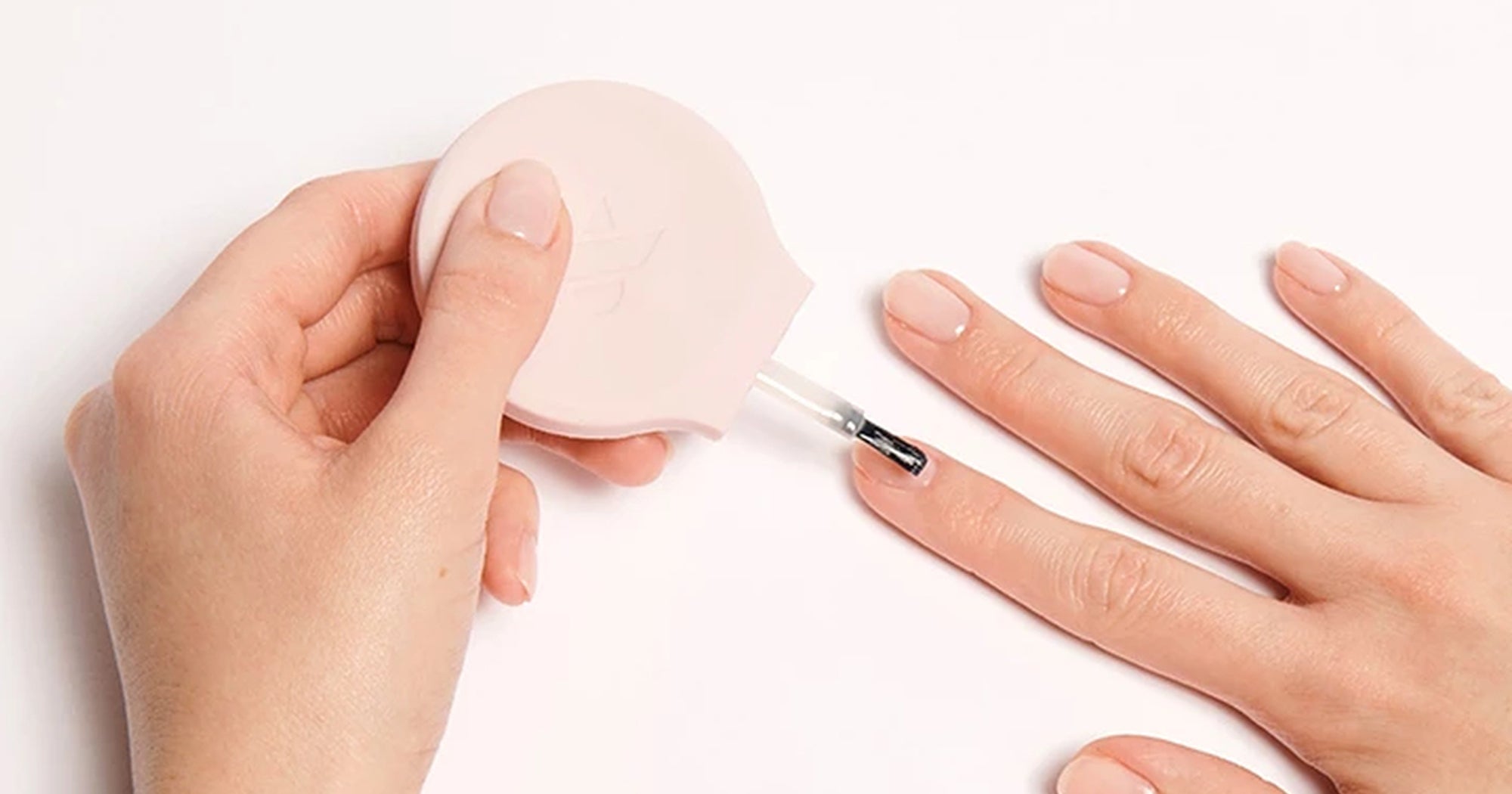In this close-up photograph, a pair of feminine hands with light skin are depicted against a soft white background. The right hand is holding a large-handled, cream white nail polish brush like a pencil, carefully applying a layer of clear nail polish to the index finger of the left hand, which lies flat on a white table with fingers gently spread. The left hand displays short, rounded nails that have already been coated with the same transparent polish, showcasing a neat and pleasing manicure. The elegant composition highlights the delicate precision involved in the nail-painting process, emphasizing the femininity and care of the hands.